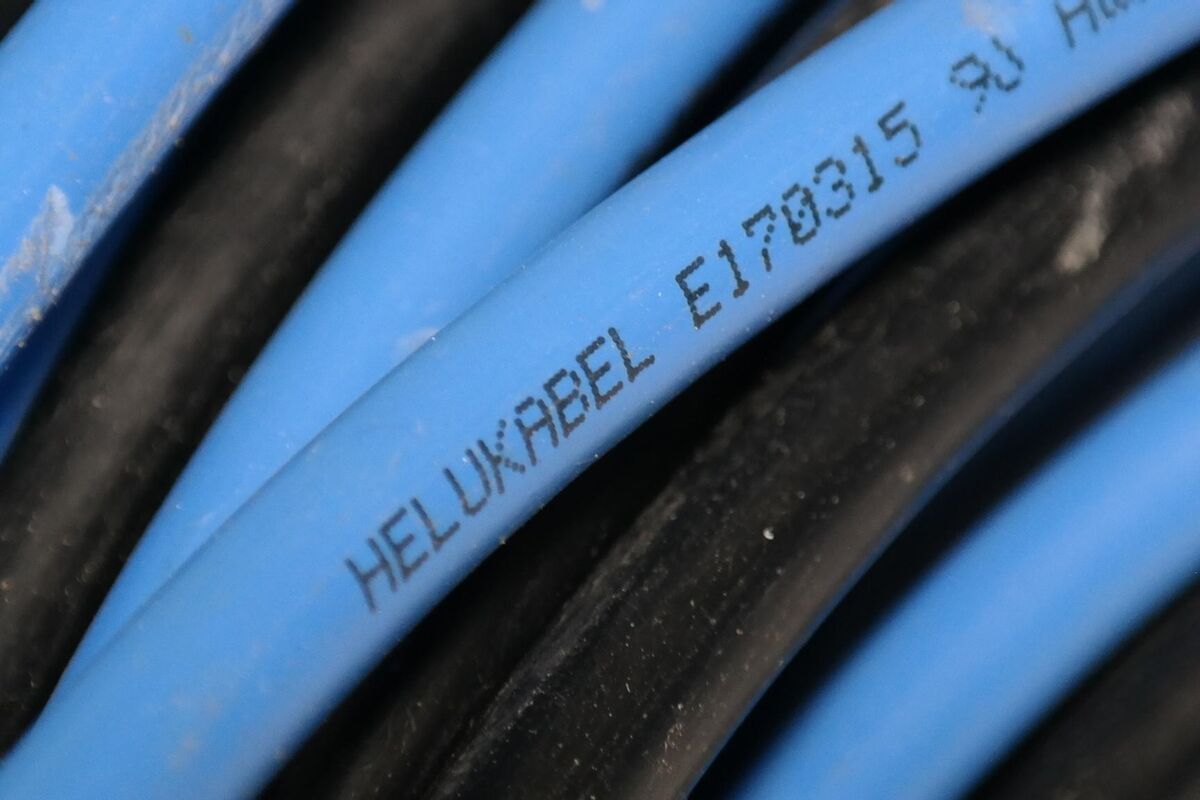This photograph captures a very close-up view of a bundle of coaxial or cable television wires. The cables are flexible but relatively thick, suggesting they could also be used for electricity. The wires are wrapped and curved around something, creating a mix of orientations from the bottom left to the top right corner of the image. Dominantly, the cables are a mixture of black, light blue, and bright blue colors. A striking feature is a light blue cable in the center, which bears black writing in thin, capitalized font that reads "HELUKABEL" followed by the identifier "E170315." There are additional characters, "9J" and the beginning of an "H," but these are cut off. The cables show signs of wear, with visible scratches and dust, indicating they are not brand new.